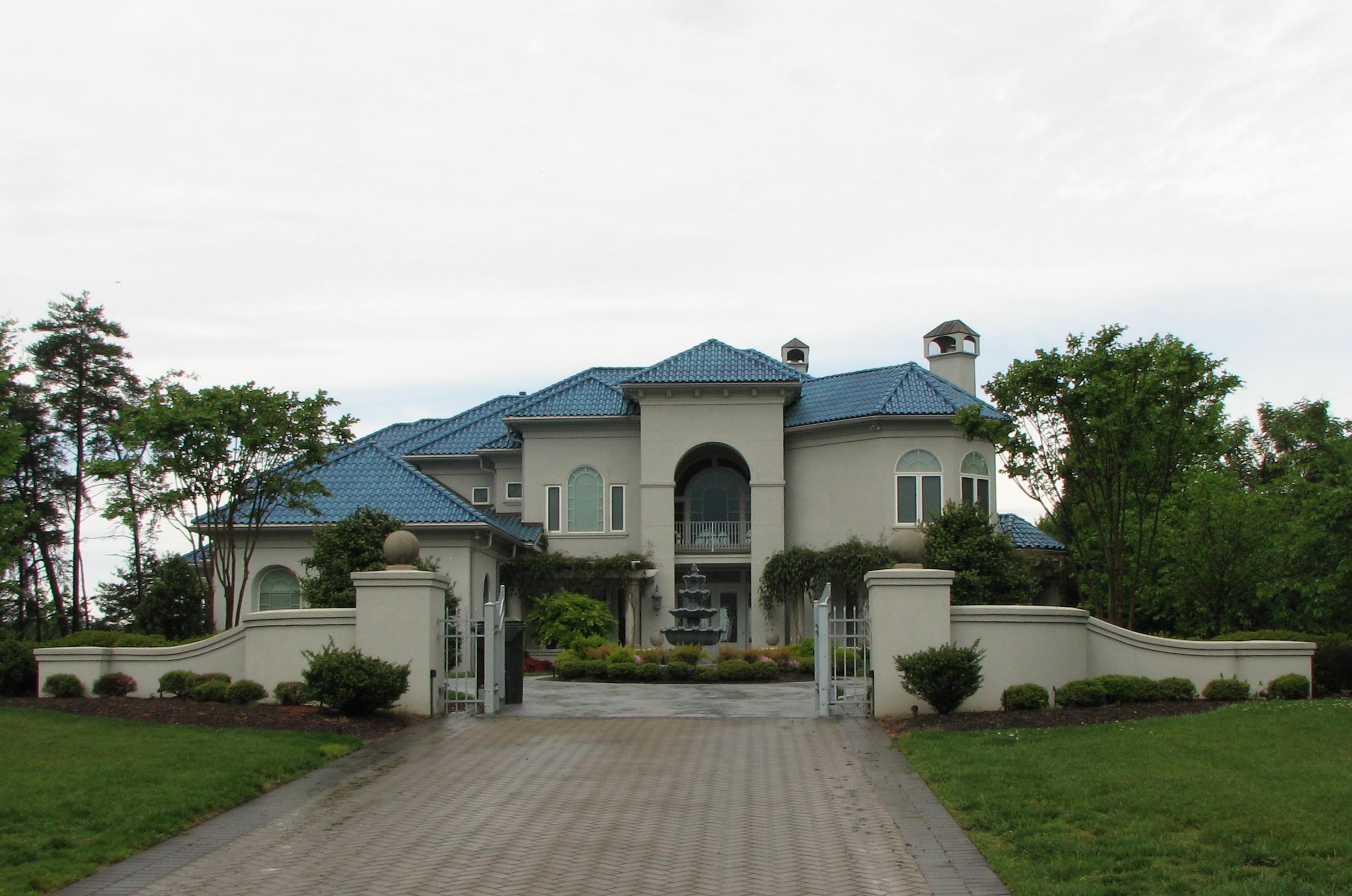The image showcases a grand, sprawling villa or bungalow, positioned prominently at the center of the scene. The photo is taken during the daytime, under a predominantly clear white sky with a hint of blue clouds peeking through. A wide, paved gray pathway leads directly to the impressive residence, bordered by neatly maintained green grass and lush gardens on both sides. On each side of the open, welcoming gate, there are two decorative pillars topped with round ornaments, with a designer guard wall extending to the left and right.

At the heart of the pathway stands an elegant, layered gray fountain, encircled by meticulously trimmed bushes and small trees. Flanking the villa are various trees, adding to the serene ambiance of the garden setting.

The villa itself boasts a sophisticated exterior in a cream-white color, accented by a distinct, blue-sloped tiled roof with multiple chimneys ascending from its peaks. The architectural design includes large windows, offering glimpses into the opulent interior, and a grand entry door framed with glass. Additionally, the upper level features a spacious balcony with a large door, providing a perfect vantage point to enjoy the surrounding landscape.

On the left side within the gate sits a smaller building, likely serving as a security post. Complementing the villa's stately appearance, the right side of the house includes two turret-like structures with open tops, enhancing the overall grandeur and elegance of the property.